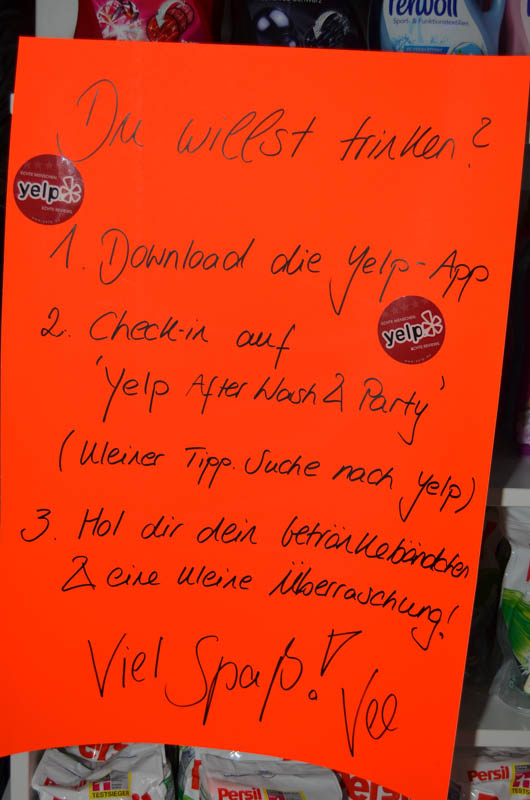The image features a photograph of a red handwritten flyer promoting Yelp, presented in both German and English. Positioned against a background containing shelves of food, including bags labeled "Persil," the flyer is crafted on orange paper stock. The flyer has three steps, each with instructions in German and their English translations:

1. "Download die Yelp-App" ("Download the Yelp app").
2. "Check in auf Yelp nach der Waschen um zu feiern" ("Check in on Yelp after you party").
3. "Hol dir dein Getränk-Beratung von Yelp" ("Get your drink recommendation from Yelp").

The flyer prominently features two red Yelp stickers, one near the top left and another in the middle right. At the bottom in larger text, the flyer encourages fun with "Viel Spaß!" which translates to "Have fun!" With carefully detailed hand-written text in black ink, the flyer aims to guide users through the process of leveraging Yelp for their social activities. The phrase "DU WILLST TRINKEN?" ("Do you want to drink?") is boldly written across the top, underlined by another Yelp sticker for emphasis.